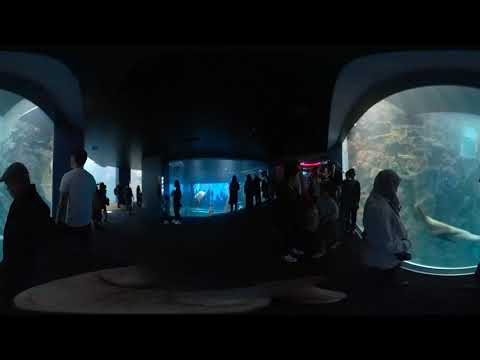The image captures a dimly-lit scene at a public aquarium, where approximately 40 silhouettes of men and women are scattered about, all drawn towards the glass enclosures that dominate the left, right, and rear sides of the room. The central area of the image is shrouded in darkness, creating a stark contrast with the illuminated tanks. The lighting from these tanks highlights the underwater environment, although the specific marine life within remains indiscernible due to the shadows. A long hallway extends into a blue-lit section of the aquarium, drawing visitors further in. On the left, a man in a white t-shirt is visible, while a girl in a white jacket stands on the right, intently observing the marine creatures. There are also a few tall cylinder structures in the middle of the room, topped with what appear to be stuffed animals, though the darkness makes it difficult to identify whether they are tigers, lions, or some other species.